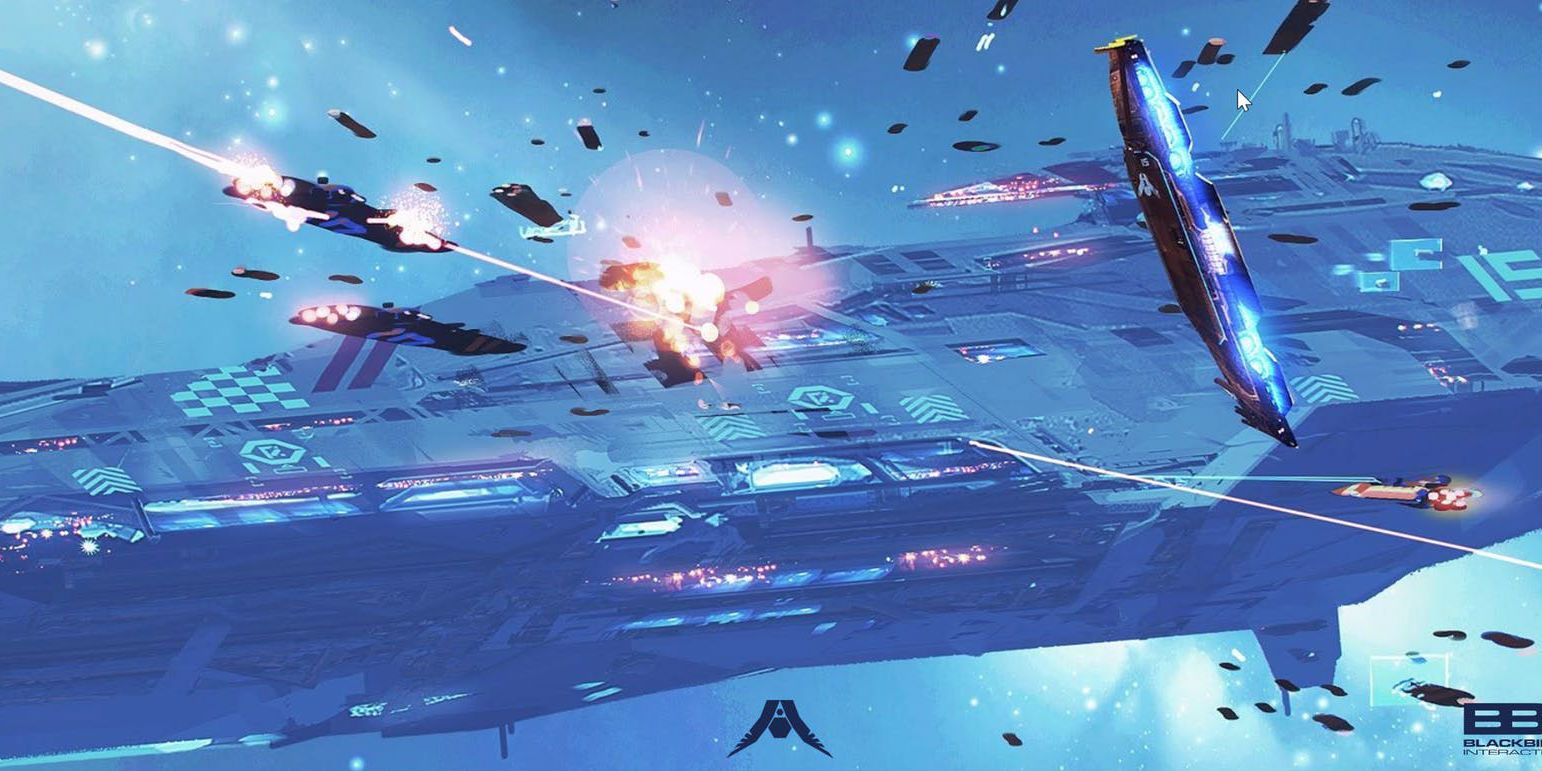The image portrays a dramatic, video game-style scene set in space, featuring an intense battle. Dominating the dark blue and black backdrop is a large spacecraft or space station, which spans the image from left to right, slightly inclining upward. The sky or space around it transitions to a lighter blue, speckled with shining stars in the upper left and lower right corners. Smaller spacecraft or aircraft, with various colored burners—some blue, some reddish-orange—are seen converging on the larger ship, launching an assault.

Exploding in the center, against the vast backdrop of the large spacecraft, is a bright yellowish-orange detonation, illuminating the scene. This explosion is marked by a white, cloudy area, with parts of the large ship flying off in all directions as black, rectangular debris. The attacking spacecraft are firing laser beams and missiles, with visible beams originating from the upper left and the bottom right, converging on the explosion. The chaotic scene is vibrant with shrapnel and lights, evoking a resemblance to the familiar, action-packed visuals of the Halo video game series.